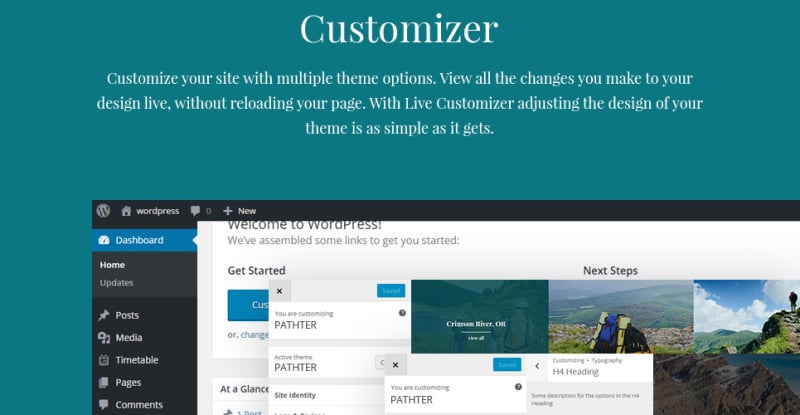On this web page designed to help users customize their WordPress site, the top section features a vibrant green background. Dominating the center are large, bold white letters that announce "Customizer." Beneath this, a subtitle explains: "Customize your site with multiple theme options. View all the changes you make to your design live without reloading your page. With Live Customizer, adjusting the design of your theme is as simple as it gets."

A prominent element on the page is a rectangle with a thick black border, noticeably thicker on the vertical sides than on the horizontal. At the top left corner of the rectangle, a circle contains a white 'W', representing the WordPress icon. Adjacent to this is a home button, and the word "WordPress" is displayed beside it. Further along the top, icons for text or chat, a plus sign, and the word "New" are visible.

The highlighted section of the sidebar menu is “Dashboard,” illuminated in blue with white lettering. Other menu options listed include Home, Updates, Posts, Media, Timetable, Pages, and Comments. Central to the page's content area, bold text greets the user with “Welcome to WordPress. We’ve assembled some links to get you started.” Below this, a call-to-action button labeled “Get Started” is present.

Several images are scattered below these instructions, featuring scenic photos such as mountains and hills. One particularly notable image shows a green overlay atop a mountain with white, albeit blurry, text, rendering the message unreadable.